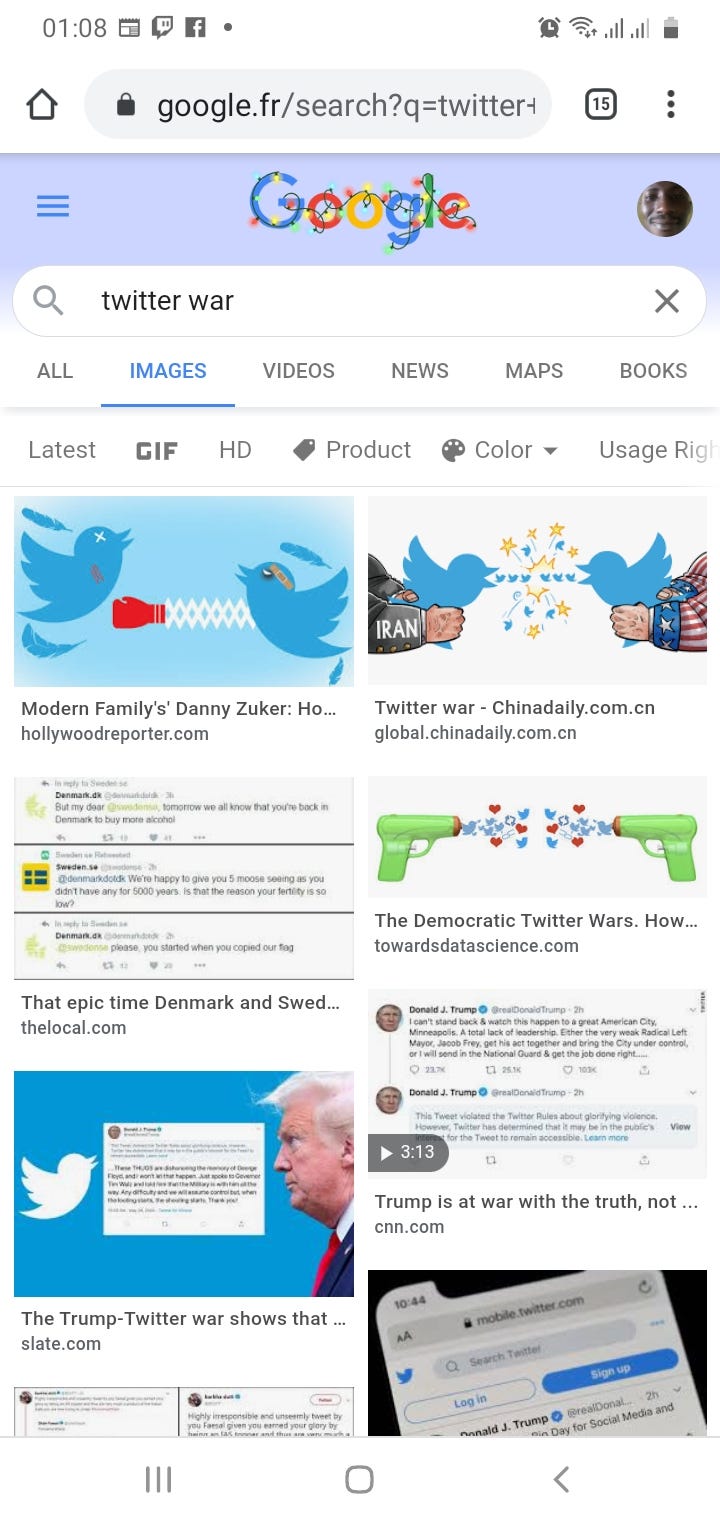This image showcases a screenshot of a Google search results page on a mobile device. The time display at the top left reads 01:08 AM. A variety of icons are visible: a news icon and a Facebook icon on the left, while the top right features an alarm icon, a Wi-Fi icon, and two network signal bars – one showing full strength at four out of four bars and the other showing three out of four. Additionally, a battery level indicator is present without a percentage rating. The browser indicates there are 15 tabs open, as seen by the Home button in the browser interface.

In the search field, the query "Twitter World" is displayed. The search categories available include All, Images, Video, News, Maps, Books, Latest, GIF, HD, Product, Color, and Usage Rights. The first search result appears to be related to "Modern Family's Danny Zuker" from hollywoodreporter.com.